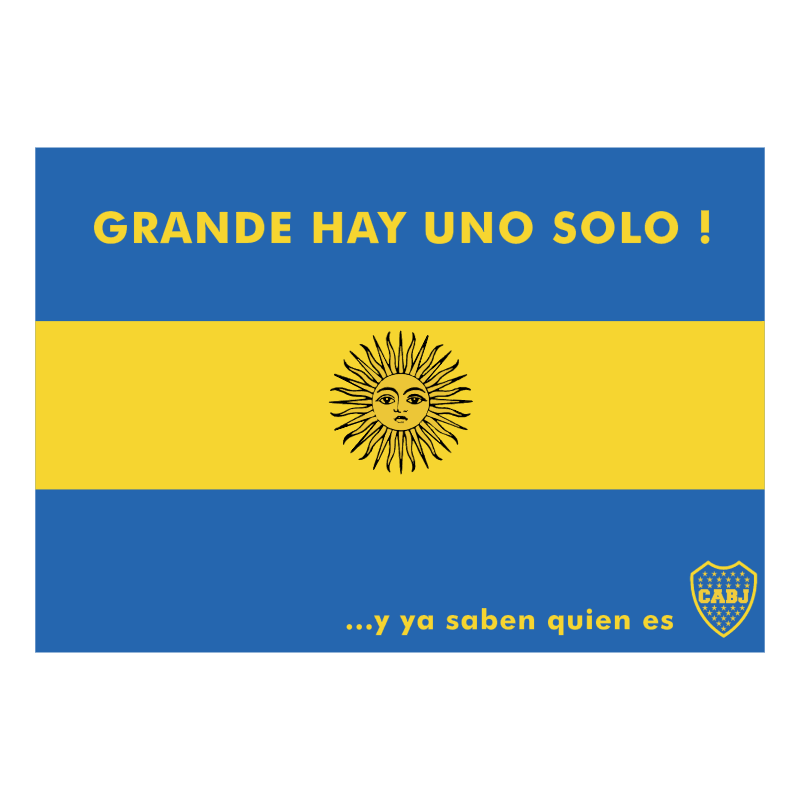The image appears to be a flag-like design, divided vertically into three equal sections with a blue-yellow-blue color scheme. At the top, in bold yellow capital letters, it reads "GRANDE, HAY UNO SOLO!" Intricately illustrated in the middle yellow section is a sun with human-like facial features, including wide eyes, arched eyebrows, a nose, and a small mouth, surrounded by approximately 25 to 30 rays, some of which are spiky while others are wavy. In the lower blue section of the image, the text "...Y YA SABEN QUIÉN ES" is displayed in yellow lettering. Additionally, a shield-shaped logo is located in the lower right corner, featuring a blue background, numerous yellow stars, and the letters "C-A-B-J" prominently positioned at its center.